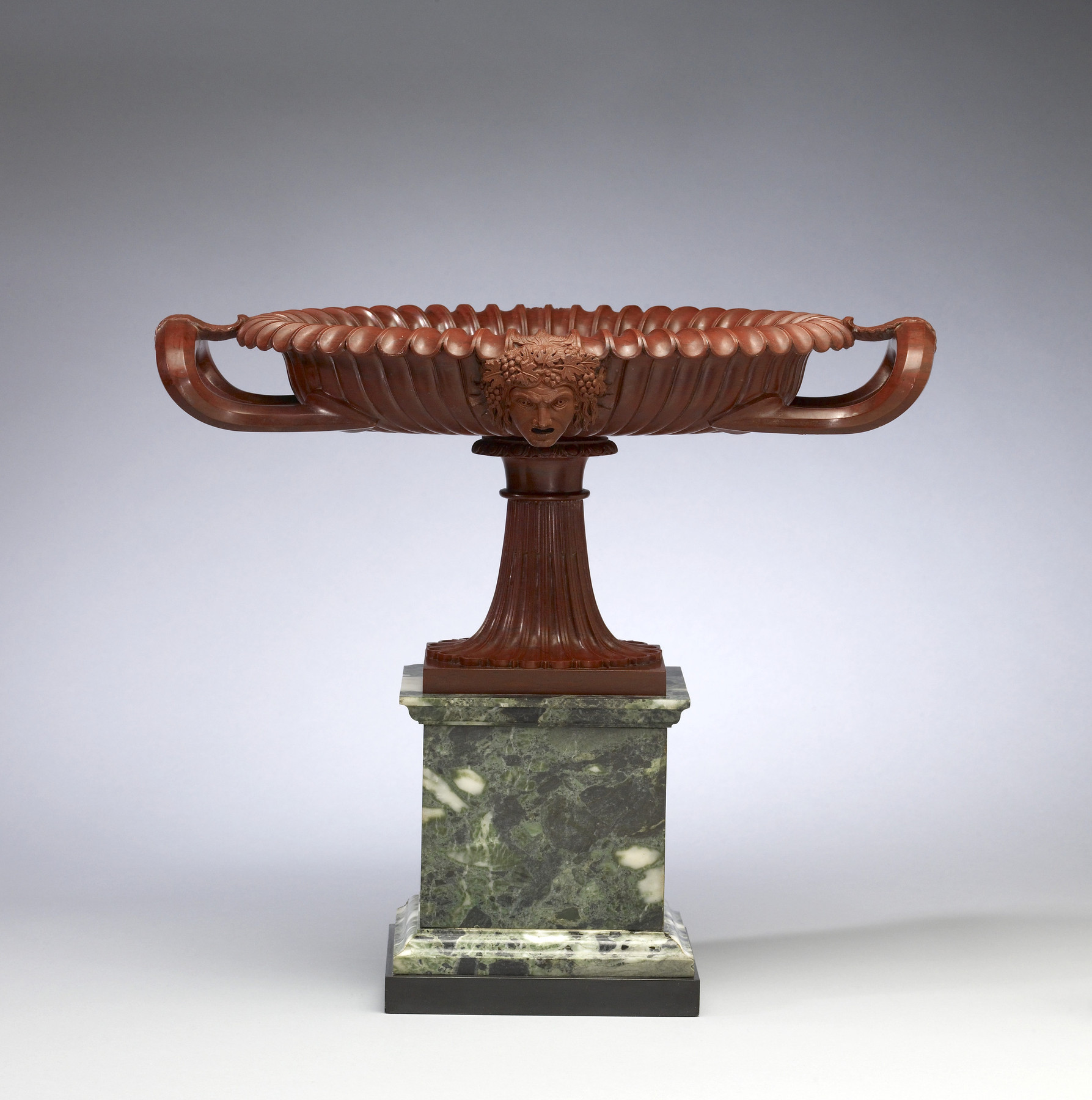The image features a highly detailed digital photograph of a unique sculpture resembling a trophy or glorified goblet. The sculpture is crafted from brown wood and features a shallow, goblet-like cup with two handles on each side. A carved human head adorns the lip of the cup, adding an intricate artistic element. The goblet is mounted on a green marble base, giving it a distinguished appearance. The entire piece rests on a light green surface, which contrasts subtly with the solid light gray background, contributing to the composition's modern and clean aesthetic. The colors in the image primarily include shades of brown, green, white, and black, highlighting the sculpture's elaborate design.